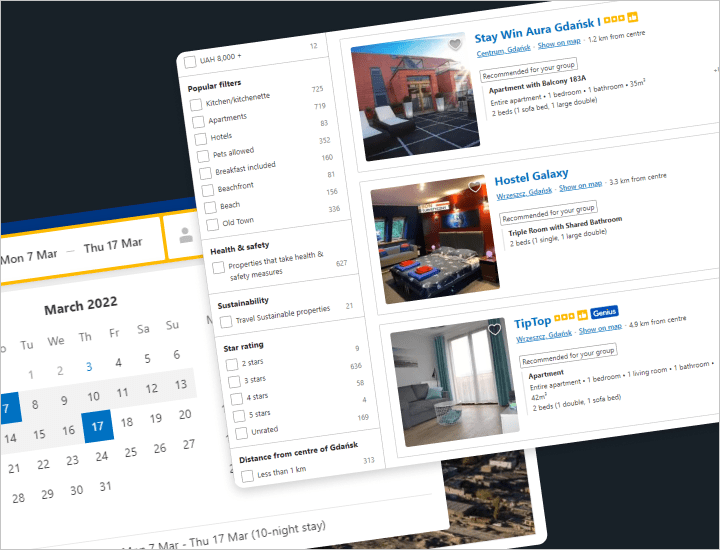The image is a screenshot of an advertisement featuring two web pages set against a black background, arranged diagonally. The upper web page is positioned from the upper right, pointing diagonally toward the lower left. This web page is dedicated to searching for apartments and hotels. 

On the left side of the page, there is a vertical list with clickable squares for applying search filters. Titled "Popular Filters," the list includes options such as Kitchen, Kitchenette, Apartments, Hotels, Pets Allowed, Breakfast Included, Beachfront, Beach, and Old Town. 

Below this section, there are additional headers including "Health and Safety" with properties that implement health and safety measures, followed by "Travel Sustainable Properties." 

Further down, there is a star rating system allowing users to select 2, 3, 4, or 5-star properties, as well as unrated ones. The final filter listed is "Distance from the center of Gdansk," indicating that the searched location is likely Gdansk, Poland. On the right side of the page, there are thumbnail images of various accommodation options available for selection.